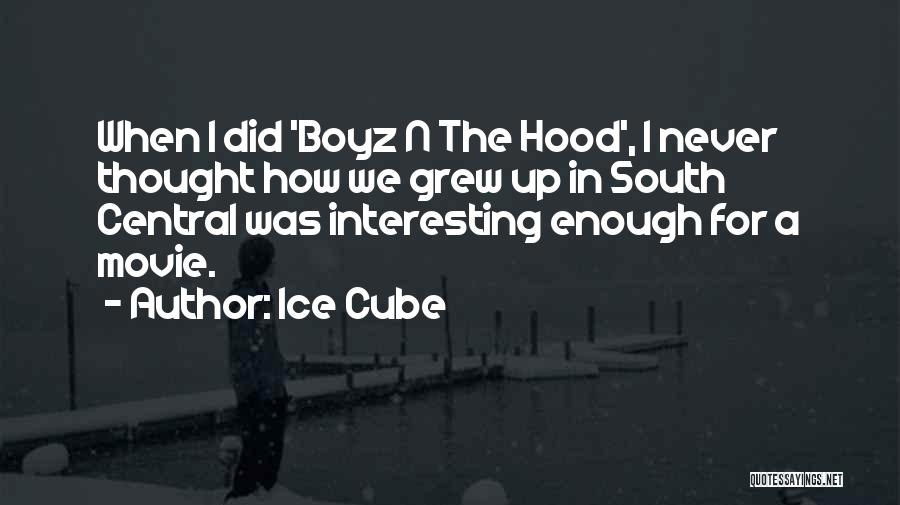The image features a poignant quote by Ice Cube superimposed on a black-and-white photograph that serves as an evocative backdrop. The quote, centered in the image with clear white font, reads, "When I did Boys in the Hood, I never thought how we grew up in South Central was interesting enough for a movie" - Ice Cube. The background showcases a younger man standing contemplatively on a snow-covered dock, gazing out over a serene, yet snow-laden lake. The entire scene is grayed out, giving it a subdued, almost introspective atmosphere, enhancing the quote's impact. Adding to its authenticity, the bottom right corner features the logo "quotessayings.net," indicating the source of the image. The quote and image together create a striking visual that emphasizes reflection and the unexpected resonance of life experiences.